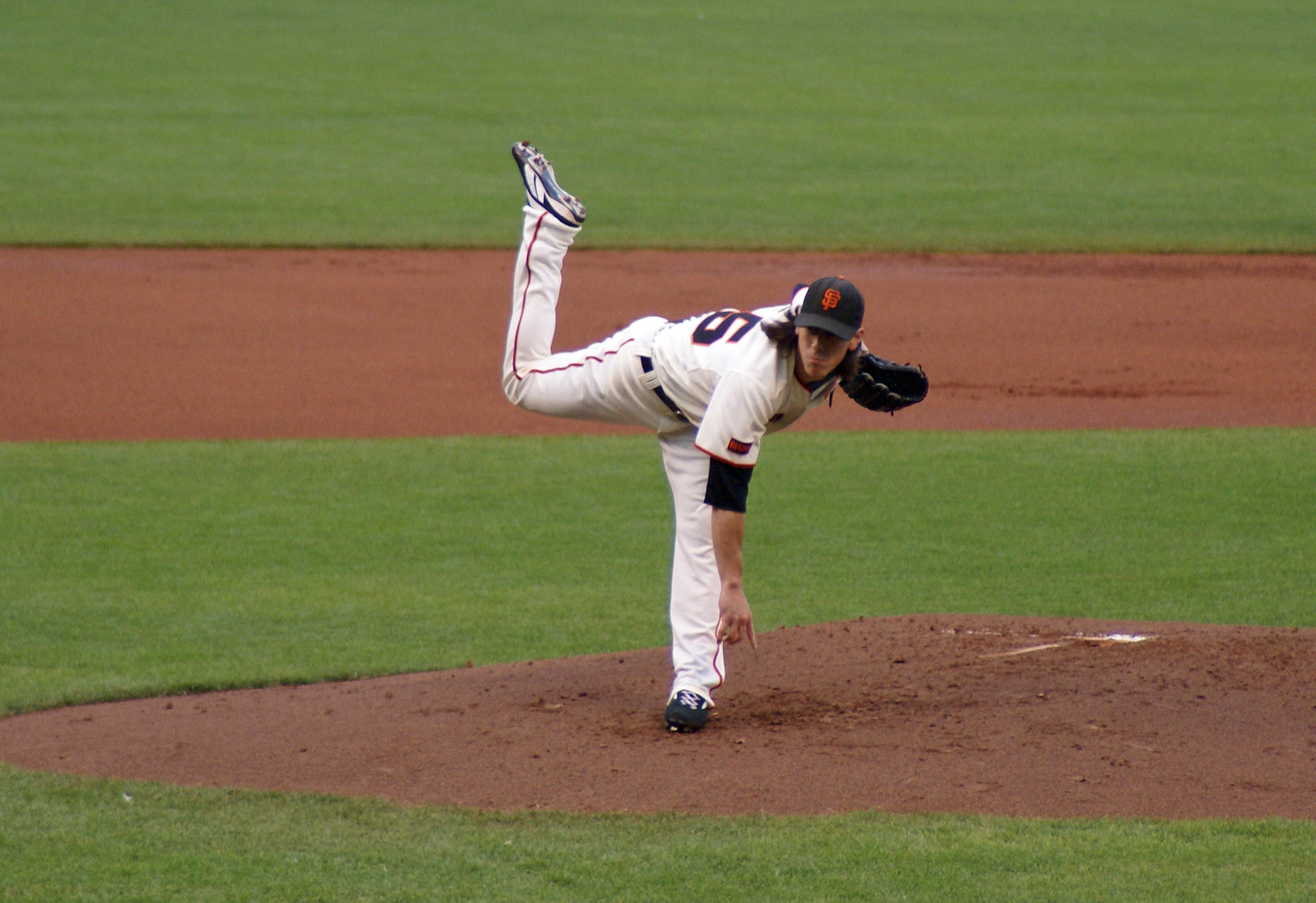In this image, we see a San Francisco Giants pitcher who has just delivered a pitch from the mound. The pitcher is in mid-motion with his right arm extended downward, almost reaching his left toes, while his black-gloved left hand is positioned next to his face. His right leg is bent at a sharp 90-degree angle, giving the impression of a powerful throw. He is dressed in the Giants' white jersey with an orange number six visible on the back, and a distinct orange stripe running down the leg of his pants. He sports black cleats, a black belt, and a black hat with the iconic orange "SF" logo. The scene takes place on a daytime baseball field, with the brown dirt mound worn and marked by usage. The baseline, also made of dirt, shows signs of runner activity, while the well-maintained green grass of the outfield and surrounding areas contrasts against the dirt. The photograph captures the athlete in dynamic action, showcasing the classic elements of baseball.